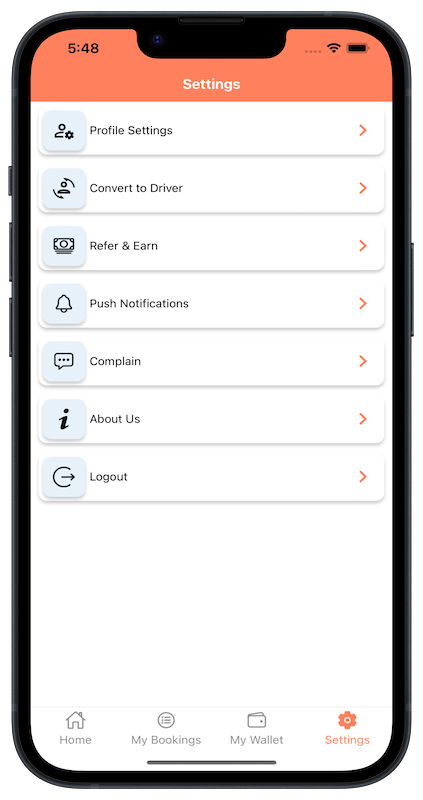Screenshot of an iPhone Settings Screen

Time: 5:48 PM
Location: Top orange header bar
Icons: Wi-Fi, Battery

Header:
- Title: "Settings" (White Text)

Main Settings List:
1. Profile Settings (Icon, Arrow)
2. Convert to Driver (Icon, Arrow)
3. Refer and Earn (Icon, Arrow)
4. Push Notifications (Icon, Arrow)
5. Complain (Icon, Arrow)
6. About Us (Icon, Arrow)
7. Logout (Icon, Arrow)

Bottom Navigation Bar:
- Home (Highlighted, Icon)
- My Bookings (Icon)
- My Wallet (Icon)
- Settings (Highlighted in Orange, Icon)